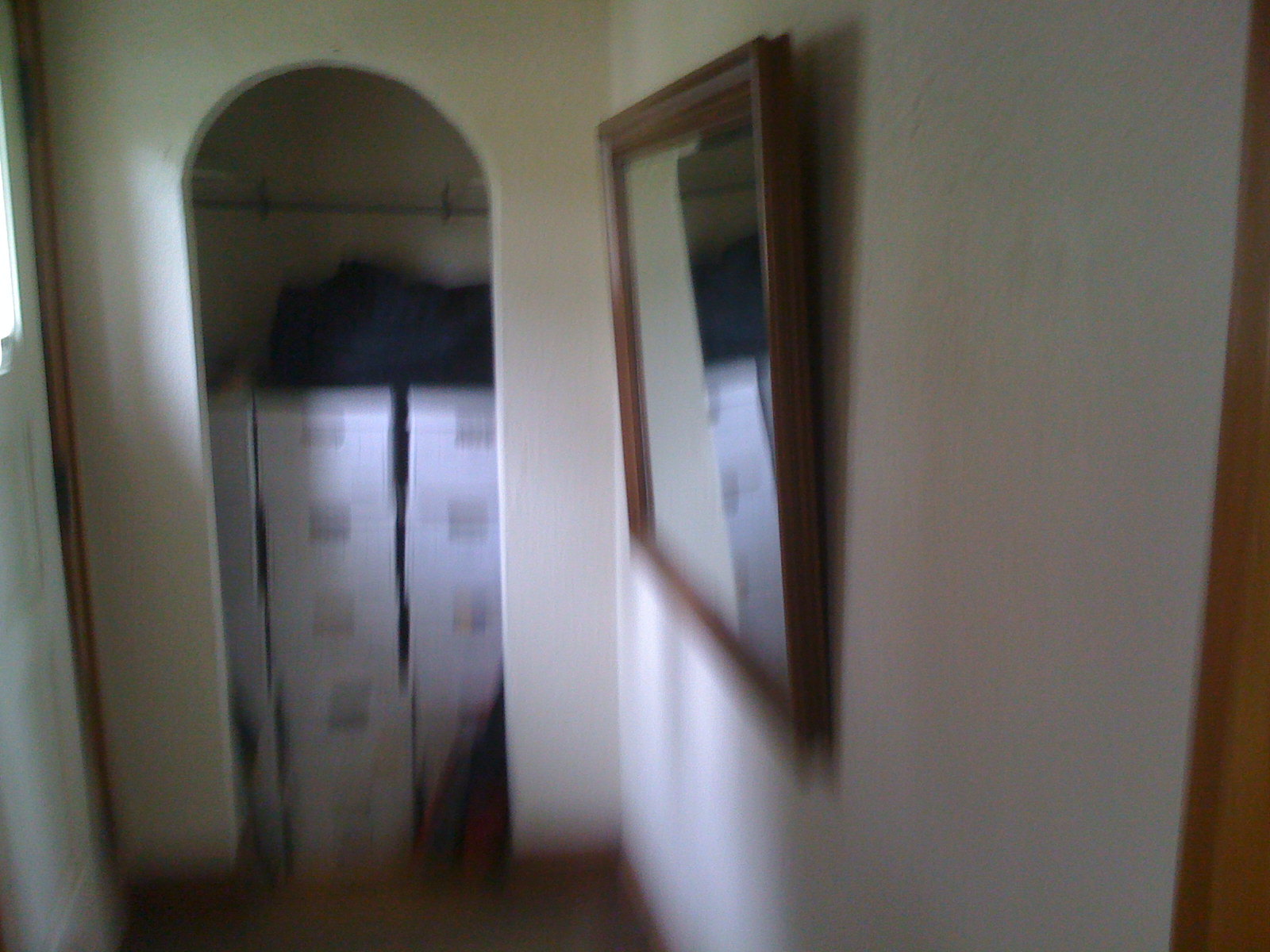The photograph captures a slightly blurry hallway scene. On the left side of the image, an off-white to pale tan wall is visible, adorned with a large, mid-tone wood-framed mirror. The mirror's expansive glass surface reflects light, contributing to the room's illumination. On the right side, a white door with a window cut-out stands, allowing sunlight to filter through and cast reflections on both the wall and the mirror. Between the mirror and the door, a narrow archway leads into a closet. Inside the closet, a dark-colored rod is mounted to the wall, supporting several stacked white cardboard boxes. Atop the boxes rests an object resembling a black duffel bag.